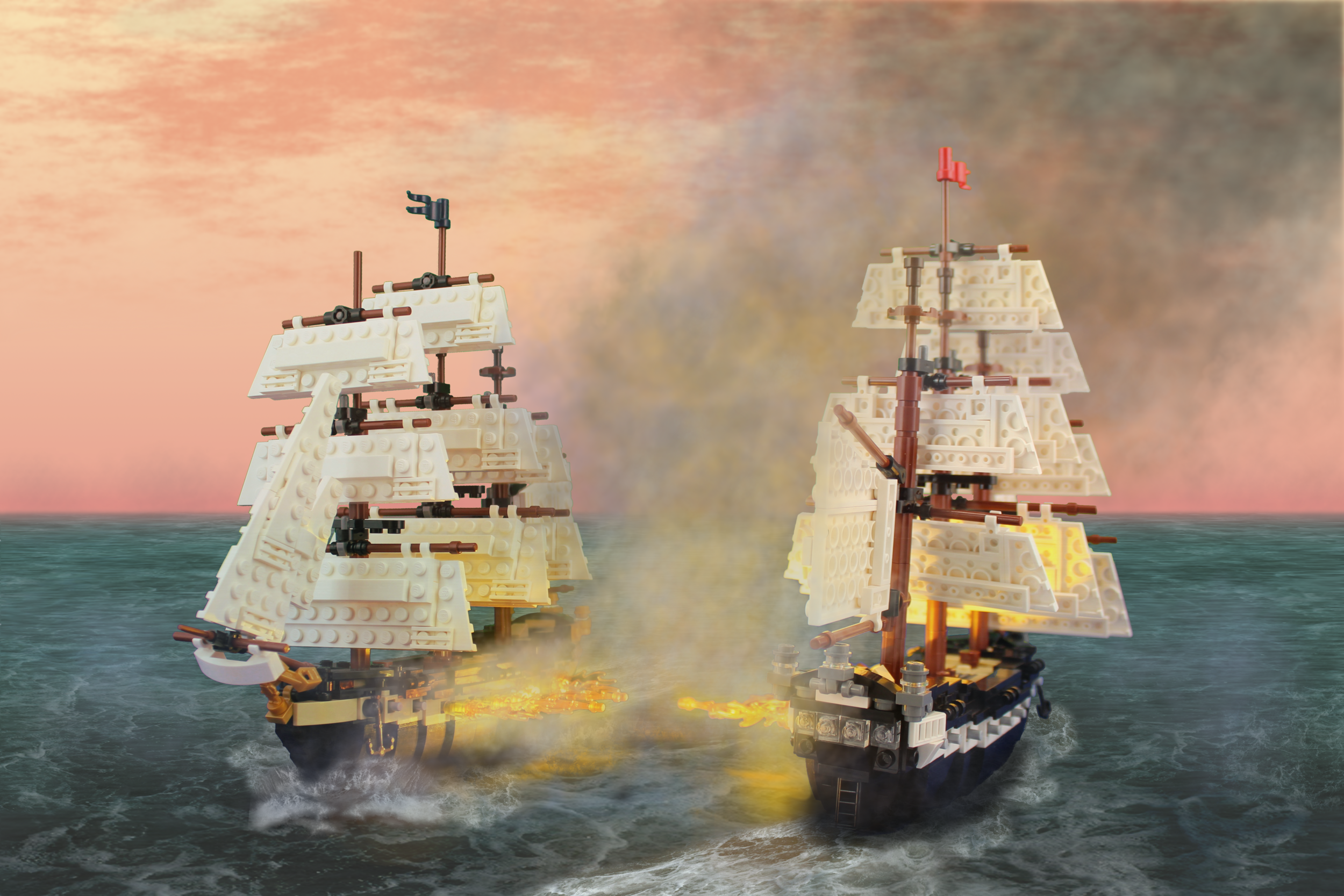This painting is a horizontally aligned rectangular artwork featuring two Lego-themed ships engaged in a naval battle on an ocean with dark grayish-blue waves. The background sky is a vibrant pink with feathery pink and white clouds. Both ships have black bodies and white sails, designed to resemble Lego pieces. The masts are also depicted as being constructed from Legos. The ship on the left flies a black flag atop a brown pole, while the ship on the right has a red flag on a similarly colored pole. Between the two ships, explosions and yellow fire effects illustrate the cannon fire exchange. Small Lego figures can be seen on the edges of the ships, adding to the intricate detail of this unique scene built entirely from Lego pieces.